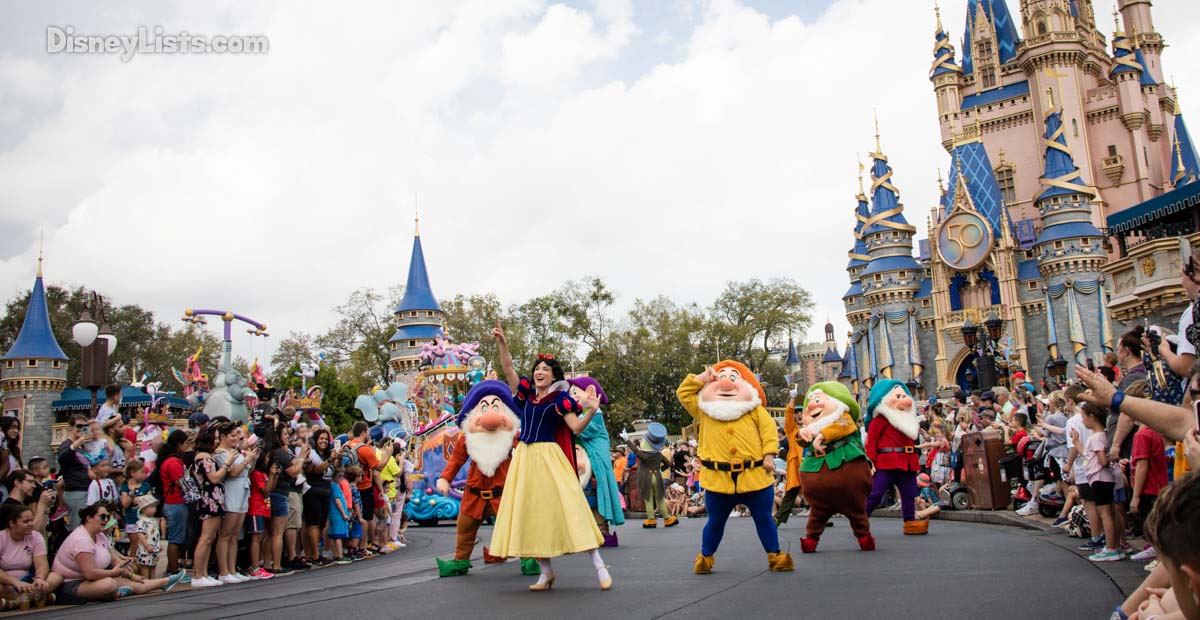The image captures a lively scene at Disneyland, with a large crowd gathered in front of the iconic beige-ish pink Cinderella's Castle, adorned with blue, pointy rooftops and a "50" emblem celebrating Disney World's anniversary. Under a very cloudy sky, Snow White, dressed in her classic blue, red, and yellow gown, performs alongside people costumed as the Seven Dwarfs, though only five—Grumpy, Dopey, Sleepy, and two others—are visible. The performance takes place on Main Street, surrounded by numerous onlookers, including many children, women waving at the characters, and people seated and standing, engrossed in the show. The upper left corner of the image features the text "DisneyList.com," and in the background, a few shortcuts are visible among a group of trees.